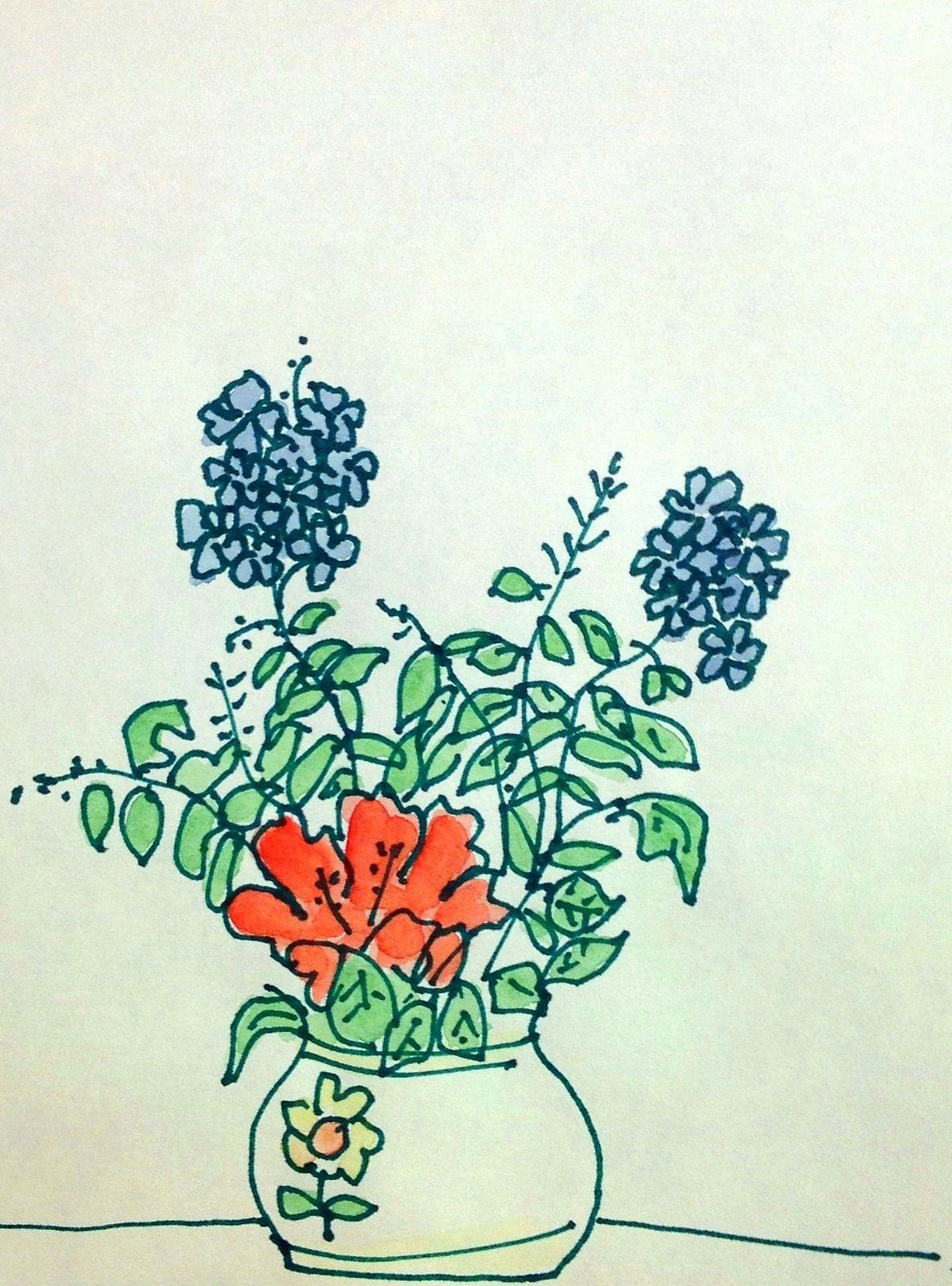A beautiful watercolor and marker illustration on off-white paper, depicting a charming arrangement of flowers in a vase. The composition is dominated by two tall, bluish-purple flowers, each boasting multiple small blooms on a single stem, complemented by green leaves at the lower sides. Nestled beneath these are clusters of ivy leaves, adding a lush, verdant texture without blossoming. At the base of the arrangement sits a large, vibrant red flower with two elegant tendrils branching out. This striking bloom is accompanied by leaves that gracefully curl over the top of the vase. The vase itself is cylindrical with gently bulging sides and features a painted yellow flower with an orange center, along with a stem and two leaves. The vase shares the same off-white hue as the paper, blending seamlessly into the background while providing a delicate canvas for the floral display.